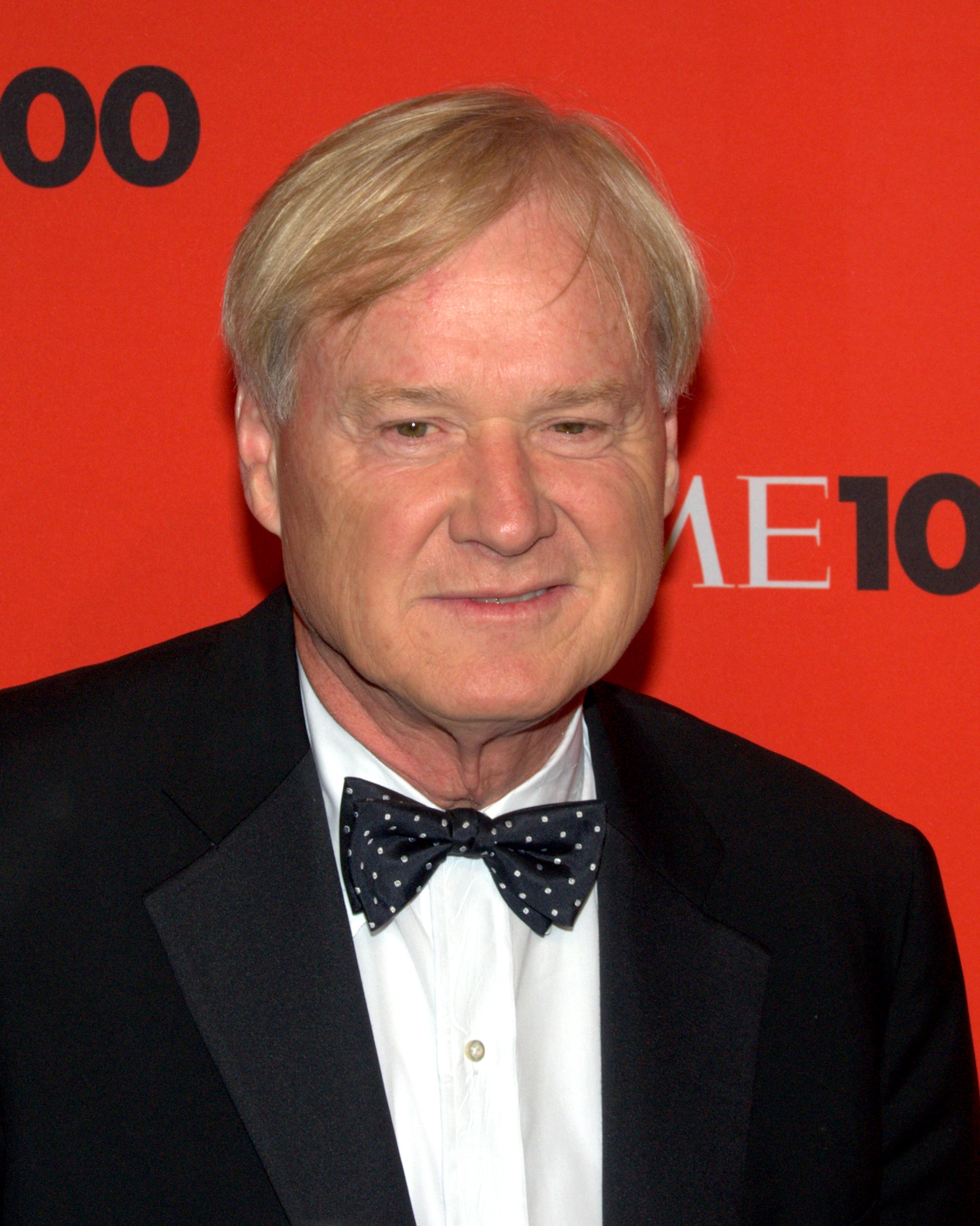The image features a close-up of journalist Chris Matthews standing in front of a vivid red background adorned with the repetitive white text "Time 100," partially obscured by his head. Matthews, captured from the chest up, is wearing a refined black tuxedo suit paired with a crisp white shirt and a distinctive black bow tie adorned with white polka dots. His blonde hair, slightly messy and parted towards the center right, frames his aging, slightly wrinkled face with hazel brown eyes. He gazes directly at the camera with a subtle smirk, seemingly during an indoor event. The contrasting colors of his attire and the backdrop highlight his presence in the center of the composition.